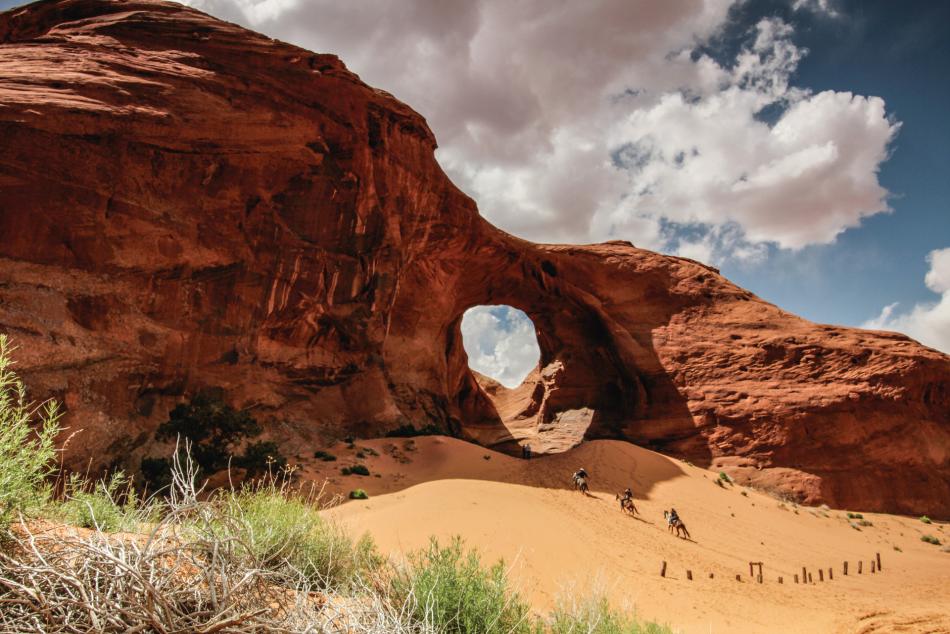The photograph captures a striking desert landscape dominated by a massive, reddish-brown rock arch that spans the entire width of the image. This grand rock formation features a central hole, resembling a naturally carved door, through which fluffy white clouds and a blue sky peek through. The arch structure is set against an uneven, sandy terrain that varies in elevation and is adorned with light golden brown hues. A touch of green vegetation—plants or bushes with light green leaves—provides contrast in the lower foreground. Adding life to the scene, three people on horseback can be seen slowly ascending the sandy slope toward the inviting archway. The sky above is filled with large white and gray clouds, casting a dramatic backdrop to this beautifully rugged landscape.